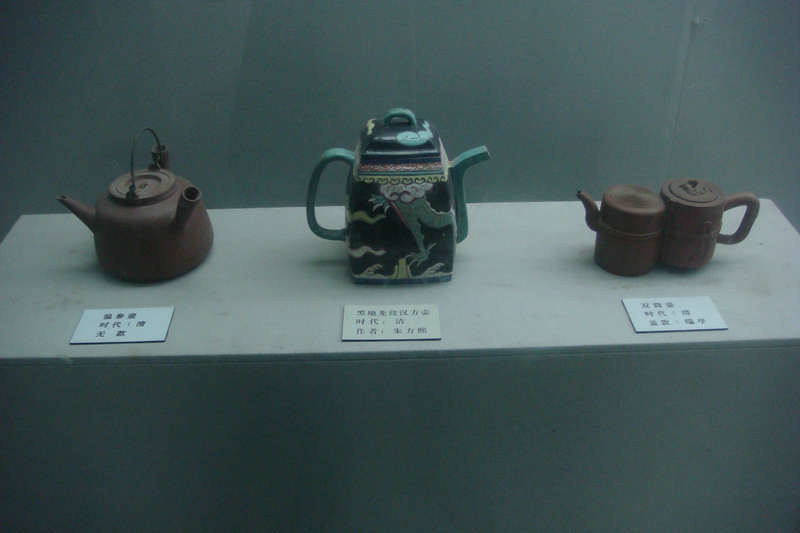This color photograph captures a museum exhibit featuring three distinct pieces of Asian pottery. The display, set against a grayish-white surface and a similarly colored three-paneled wall, showcases these intricate teapots with accompanying placards, which feature black Asian writing—likely Chinese or Japanese.

On the left, a terracotta teapot with two spouts and a wire handle stands out. This teapot seems to be designed for steam release rather than pouring. The central piece is a porcelain teapot, square-shaped and painted in rich shades of dark blue with ornate designs, including those resembling mythological creatures and clouds. It also features a steam-releasing spout and a handle, suggesting a unique function. To the right, another terracotta teapot with a distinctive design resembling two conjoined barrels catches the eye. This piece houses a spout on one end and a removable lid on the section where the handle is attached. Adjacent to it is a small tea cup, completing the set.

The display, meticulously arranged, emphasizes the historical and artistic significance of these antique teapots, highlighting the cultural heritage they represent.